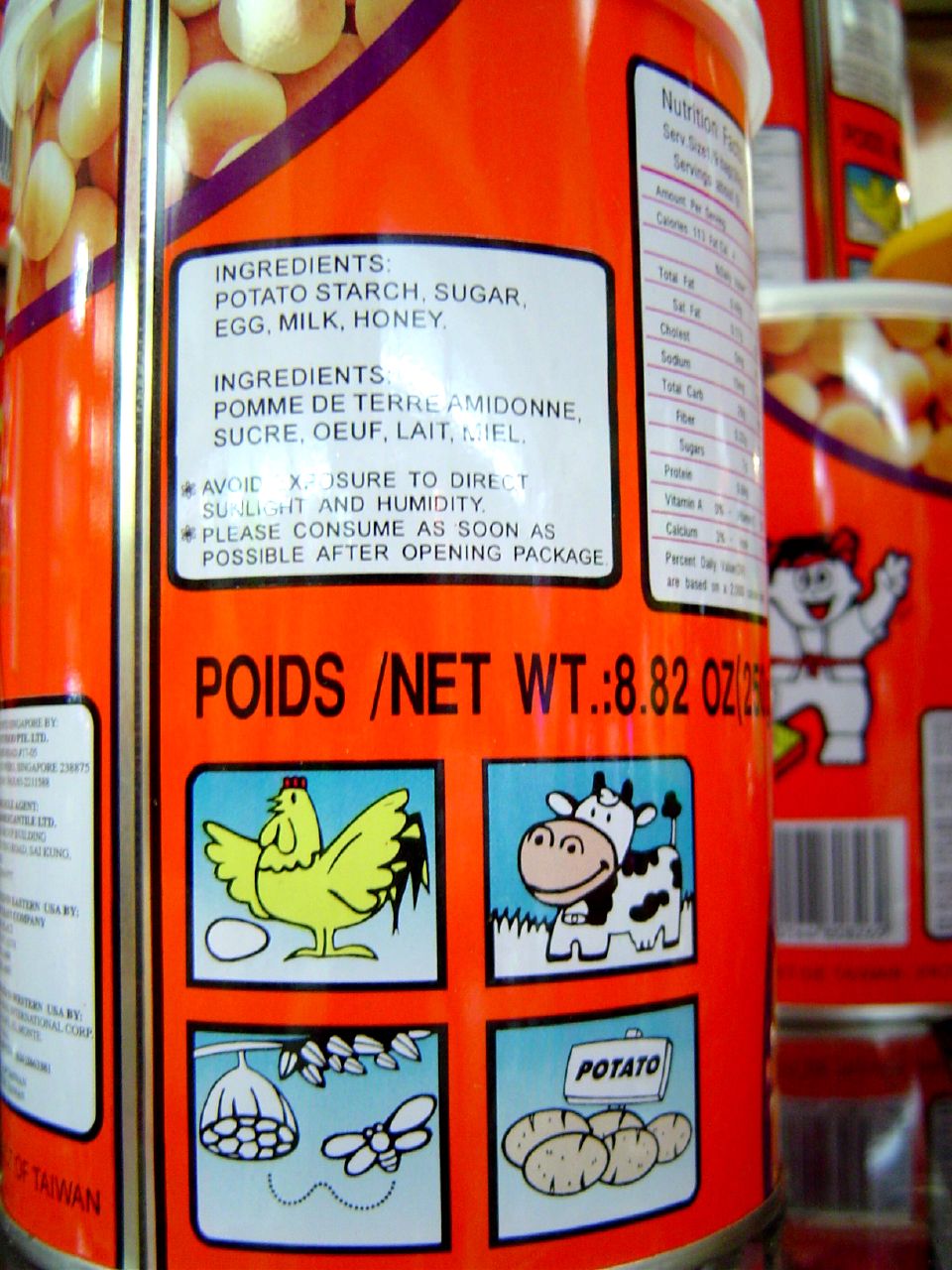This is a detailed close-up photograph of a cylindrical red tin, primarily used for snack foods, which prominently features nutritional information and pictorial illustrations. The top left corner displays a seam that runs vertically along the can. To the right of the seam, an ingredient list is provided in both English and French, stating the components as potato, starch, sugar, egg, milk, and honey. Additionally, cautionary labels advise against exposure to direct sunlight and humidity, and recommend consuming the contents promptly after opening. A white box with black lines outlines the nutritional facts, though specific values are hard to discern; however, elements like sodium, sugars, protein, vitamin A, and calcium are mentioned.

The tin boasts a series of small square illustrations on a blue and white background. These include a yellow chicken with black tail feathers and red comb standing next to a white oval egg, a white cow with black spots and peach face with black markings, a bee depicted flying between flowers, and a group of brown oval potatoes. Below these images, the net weight of the package, 8.82 ounces, is noted.

On the left-hand side of the can, towards the bottom, the word "Taiwan" is printed. The can is topped with a clear plastic lid, and a similar can, also with a plastic lid, is visible in the background, suggesting a display setup. Additionally, there is a small depiction of a young boy waving above a barcode, partially obscured but present on the can.